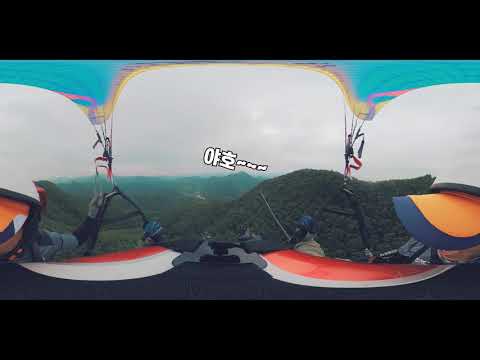The image depicts a person paragliding over a scenic, mountainous landscape. Captured through a fisheye lens, the scene offers a distorted yet immersive view from above. The colorful parasail, featuring shades of yellow, pink, teal, red, and blue, dominates the upper part of the image. Dangling cords are visible, extending upwards to the parasail. The paraglider, seen wearing a white helmet with black trim, a reflective mask with orange and red hues, and holding onto the rigging, captures a dynamic selfie. Additionally, a baseball cap with an orange and purple rim appears on the right side of the shot. In the center of the image, two Korean characters along with some dashes stand out, possibly indicating text. The extensive background reveals rolling hills transitioning from vibrant green to turquoise, under a predominantly gray, overcast sky suffused with sunlight.